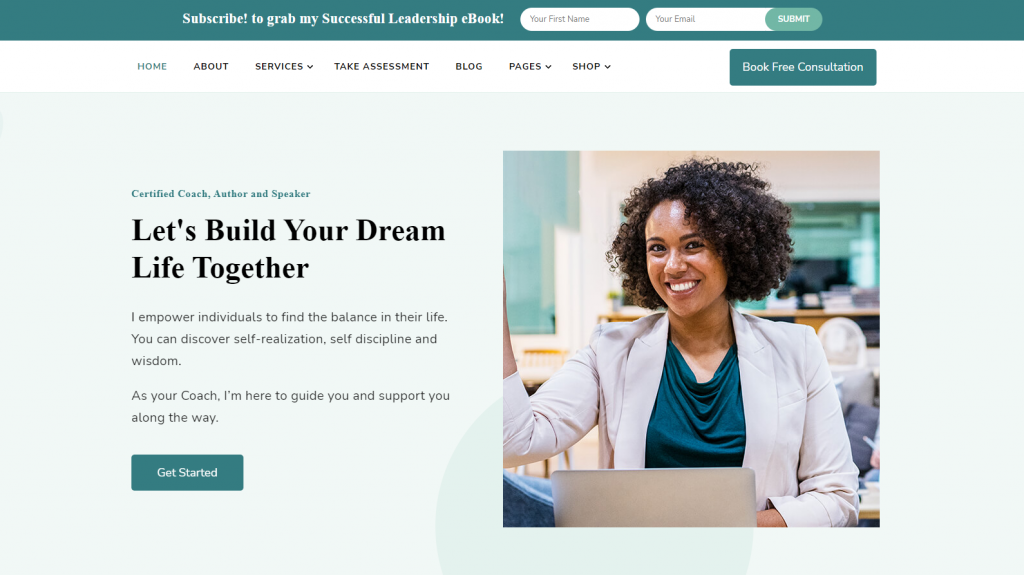Here is a cleaned-up, detailed caption for the described image:

---

The image is a screenshot of a professional self-improvement website. A dark green bar runs across the top, featuring a call-to-action in white lettering on the left: "Subscribe! to grab my successful leadership e-book." To the right, there are two white oval fields for user input, labeled "your first name" and "your email" in gray, accompanied by a gray and white "Submit" button.

Below this, there is a horizontal navigation menu starting with "Home" in light blue font, followed by "About," "Services," "Take Assessment," "Blog," "Pages," and "Shop" in black font. On the far right side of the menu is a long rectangular green banner with white text that reads "Book Free Consultation."

The main content area is slightly off-white. At the top, in green text, it reads "Certified Coach, Author, and Speaker." Below this, in bold black lettering, it says, "Let's build your dream life together." The accompanying text states, "I empower individuals to find the balance in their life. You can discover self-realization, self-discipline, and wisdom. As your coach, I'm here to guide you and support you along the way." At the bottom left is a rectangular green button labeled "Get Started" in white text.

On the right-hand side of the screen, there is a large image of a young woman in her early 30s. She is wearing a white blazer and a dark green top, and is smiling. The top of her laptop is visible at the bottom center of the image, giving the impression that she is engaged in her work or a digital consultation.